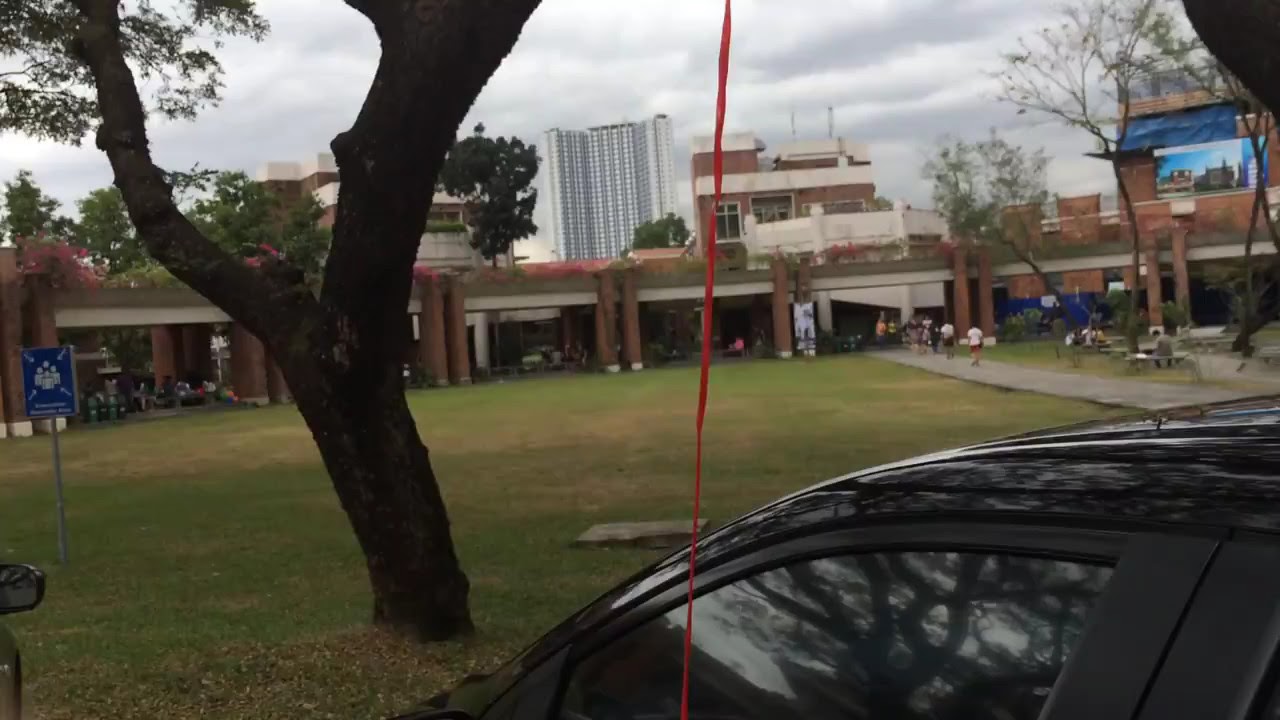The image depicts a bustling outdoor scene on what appears to be a school or campus ground set in a downtown area. Central to the image is a large grass field bordered by a brick archway that surrounds the entire grassy area, providing a picturesque, enclosed space. A pathway runs through the center of the grass field, leading directly to a prominent multi-story building in the background, which may be part of an educational institution, such as a high school or college.

In the foreground, the image includes a black car with a red antenna, seen from the perspective of someone standing right next to it. The side mirror of another vehicle is partially visible in the bottom left corner. There is a tree with bifurcated trunks adjacent to the foreground car, casting reflections on the car window, which also mirrors the image of another tree.

People can be seen walking along the pathways beneath the arch structure, enhancing the lively atmosphere. To the right is a display, potentially showcasing city information or school programs, typical of a city college. Additionally, a blue metal sign on the left features white illustrations of a group of four people and directional arrows, possibly indicating the school's logo or a designated meeting point.

Surrounding the central field and pathway are several benches, more trees, and abundant greenery, with plants growing around the roofing of the nearby buildings. The sky overhead is heavily clouded, adding a moody backdrop to the scene. Tall buildings in the distant background further emphasize the urban setting.